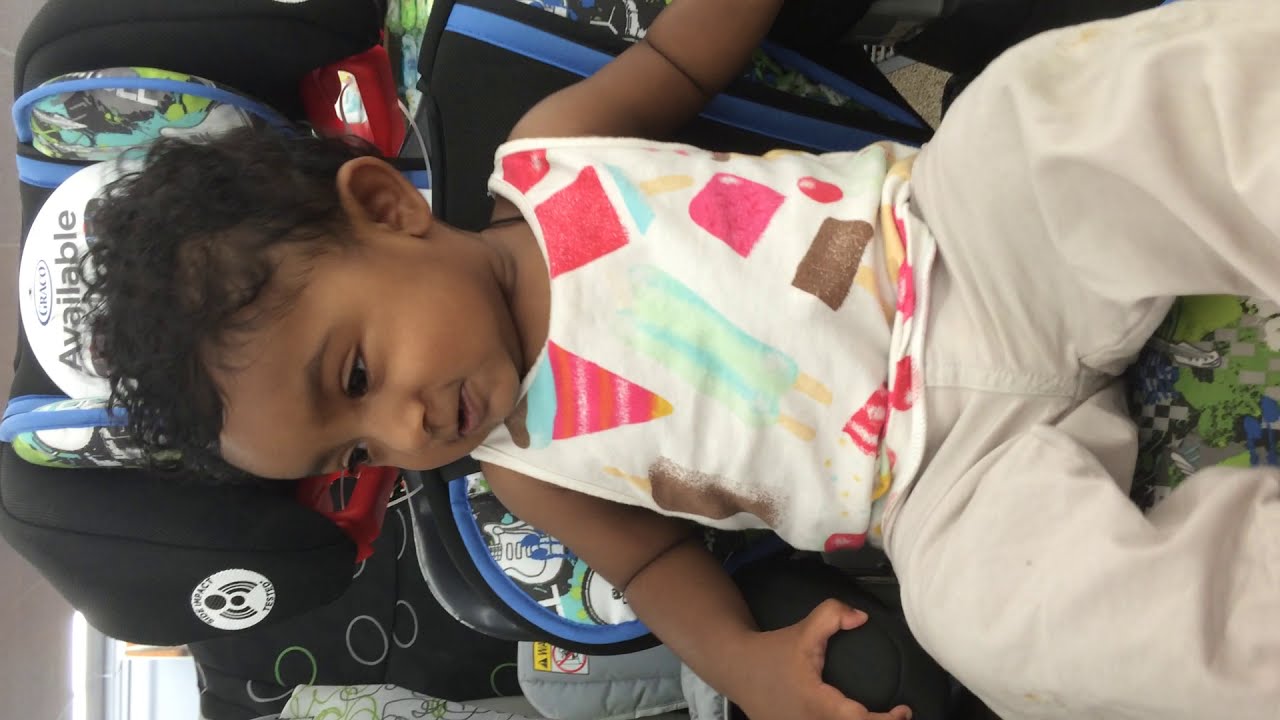The image features a young child, likely an Indian boy around one or two years old, seated in a car seat or children's chair that is turned 90 degrees to the left, requiring a head tilt to the left for a normal view. The boy, with curly black hair, is wearing a white tank top adorned with various red, blue, and brown shapes, including triangles, squares, and ice cream-like designs, matched with off-white khaki long pants or beige shorts. He has a slight, expectant smile on his face, appearing happy. His hands are gripping the armrests of the seat, which is predominantly black and blue with white and green sections. The seat features a headrest and some child-friendly character designs, though they are obscured by the child's positioning. Behind him, there is something with the word "available," suggesting that he might be on a children's ride at an event like a carnival.